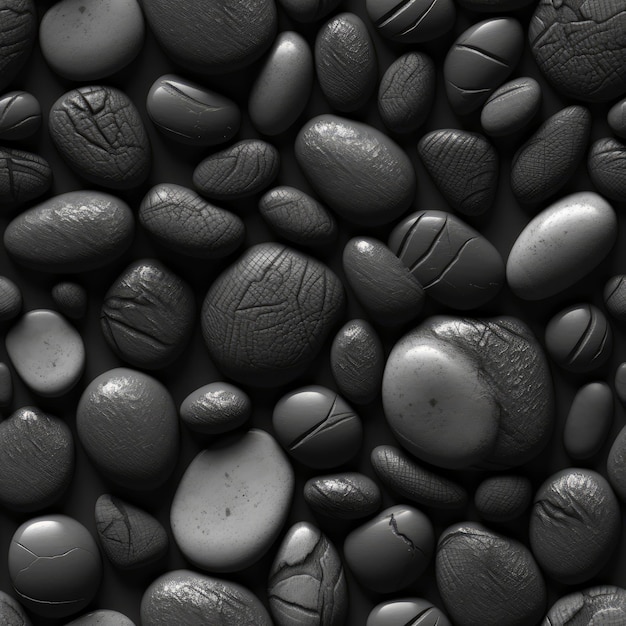The image appears to be a computer-generated black-and-white depiction of an assortment of small rocks and pebbles. The composition mimics a textured gravel collage with an array of dark gray stones of various shapes, including round, oval, spherical, bean-shaped, and pear-shaped. Each rock exhibits unique features and textures: some are smooth and shiny, others have cracks and crevices resembling reptile skin or creased leather. The diversity in texture ranges from purely smooth surfaces to dotted and deeply cracked patterns. Despite the monochrome palette, the rocks exhibit different shades of gray, from light to deep and dark, with distinct highlights that emphasize their textured surfaces. The background between the rocks is black, accentuating the contrast and making the individual stones stand out. The scene evokes the appearance of scattered pebbles one might find on a rocky beach or riverbed, arranged close together in an aesthetically pleasing manner.